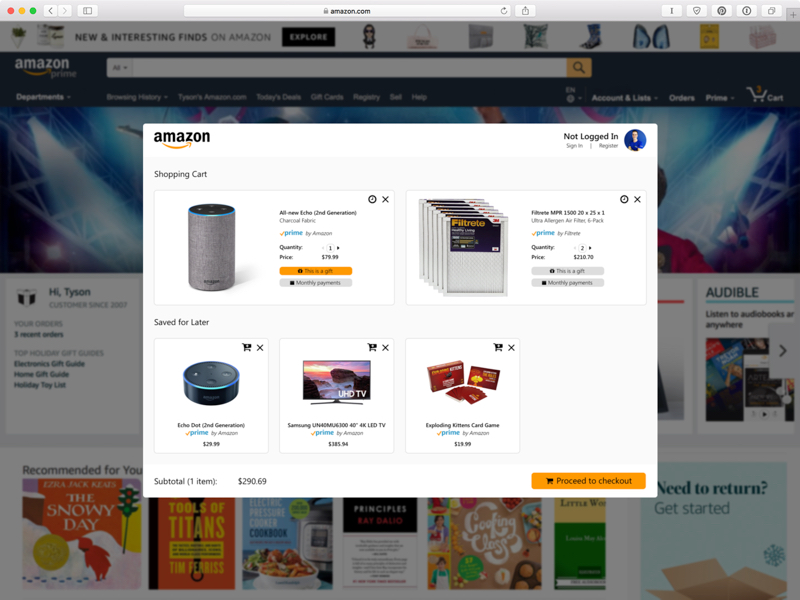This image is a detailed screenshot of the Amazon website, viewed on the Safari browser. At the very top of the screen, the Safari browser’s typical interface is visible with the red, yellow, and green circles in the top left corner for quitting, minimizing, or maximizing the window. Just beside them are back and forward navigation buttons. The URL bar shows "amazon.com", and to the immediate right, there are icons for a shield with a checkmark, an information icon, and a copy icon.

The primary focal point of the screenshot is a central pop-up or overlay against the slightly blurred Amazon homepage background. At the top of this pop-up, the Amazon logo is prominently displayed, featuring the recognizable gold arrow smile. In the top right corner of this overlay, it says "Not logged in" accompanied by a default profile photo. Directly below that, there are options to "Sign in" or "Register".

In the middle section of the overlay, the shopping cart contents are displayed. It first lists an "All-new Echo (2nd Generation)" as a selected item. To its right, there appears to be an item labeled "Filbright MFR filters," though the text is somewhat blurry and indistinct. Below these items, additional products are shown: another Echo device, a Samsung TV, and the "Exploding Kittens" card game. 

Towards the bottom of the overlay, the subtotal is noted as "1 item: $290.69". Finally, in the bottom right corner, there is a yellow rectangular button labeled "Proceed to checkout".